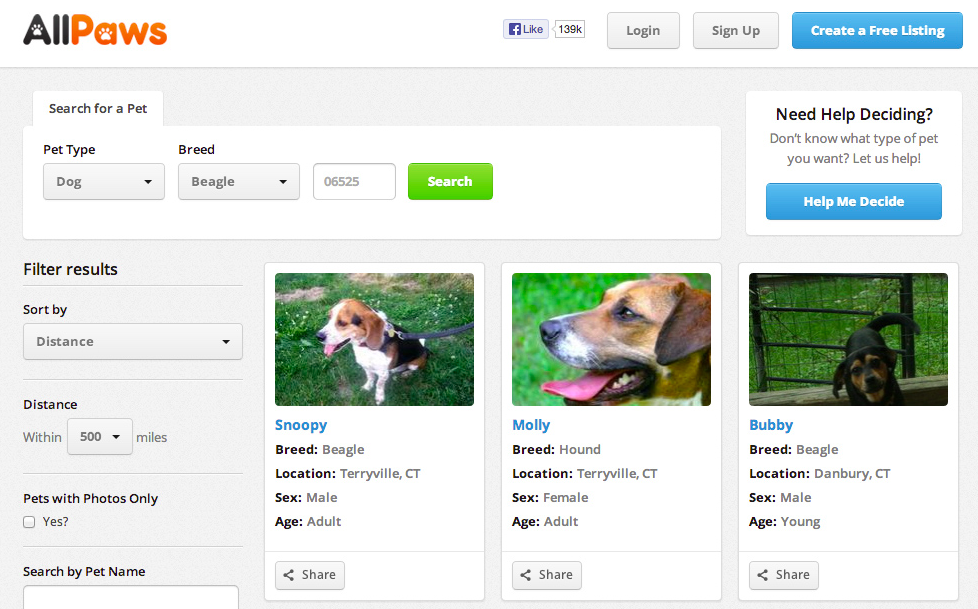The website banner prominently features the name "all PAWS," where the "all" is written in black and the "PAWS" in orange. Notably, the "A" in both "all" and "PAWS" incorporates small paw prints within the letter. Below this, the website displays three images of dogs:

1. **Snoopy**  
   - **Breed:** Beagle  
   - **Location:** Terryville, CT  
   - **Sex:** Male  
   - **Age:** Adult  
   *Image description:* Snoopy is sitting on the grass, looking alert and content.

2. **Molly**  
   - **Breed:** Hound  
   - **Location:** Terryville, CT  
   - **Sex:** Female  
   - **Age:** Adult  
   *Image description:* Molly is also on the grass, possibly at the same location, appearing calm and gentle.

3. **Bubby**  
   - **Breed:** Beagle  
   - **Location:** Danbury, CT  
   - **Sex:** Male  
   - **Age:** Young  
   *Image description:* Bubby looks playful and energetic, suitable for a younger dog.

At the top of the page, there is a search function labeled "Search for Pet," with options below for specifying "Pet Type" and "Breed" before executing the search.